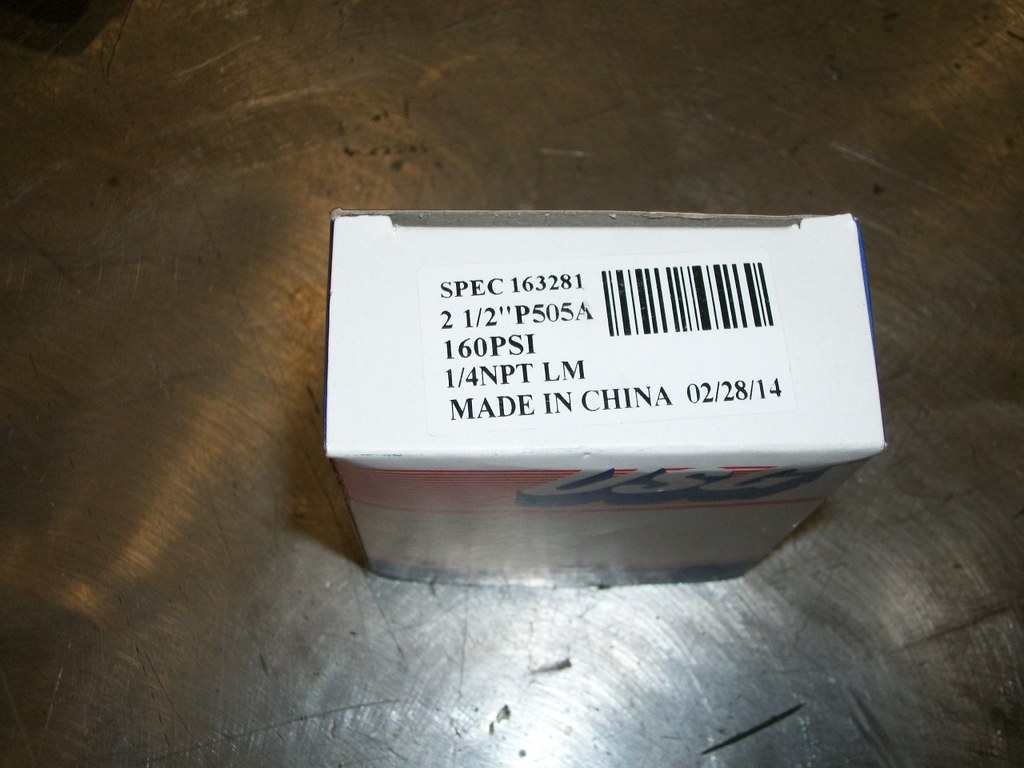The image shows a white box positioned on a steel table. The perspective allows us to view the top and the front side of the box. The top edge of the front side features a distinct orange or red band, with the acronym "USG" prominently displayed in bold, white block letters. Below this vivid strip, the box is primarily white, with a blue line running near the bottom edge. On the top surface of the box, a barcode is prominently visible alongside detailed product information. The text reads: "SPEC 163281, 2.5 inch P505A, 160 PSI, 1/4 NPT LM, made in China, 022814."